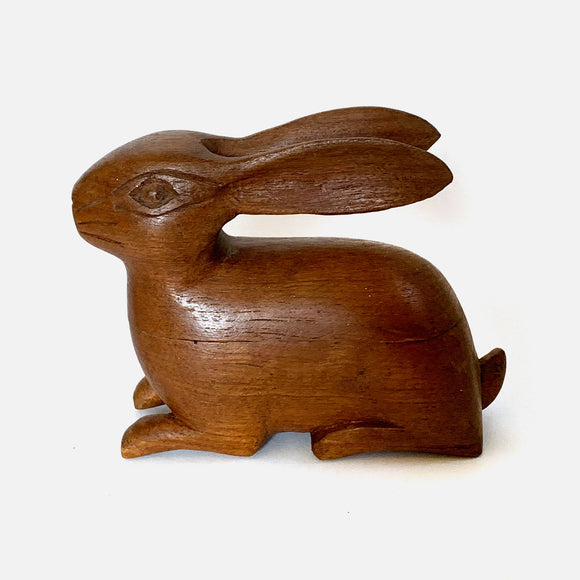This is a detailed image of a simple hand-carved wooden bunny rabbit figurine set against a solid white background. The dark brown varnish gives the figure a polished finish. The bunny is captured in profile, sitting with its legs bent at an angle, facing towards the left side of the picture. The ears are pointed backward toward the right side. The face features an eye with an oval outline and a few carved whiskers that give the bunny a somewhat skeptical or angry expression. Additionally, there is a small, upwards-pointing tail completing the figure. The carvings skillfully highlight each part of the bunny's body, making it a cohesive and intriguing wooden sculpture.